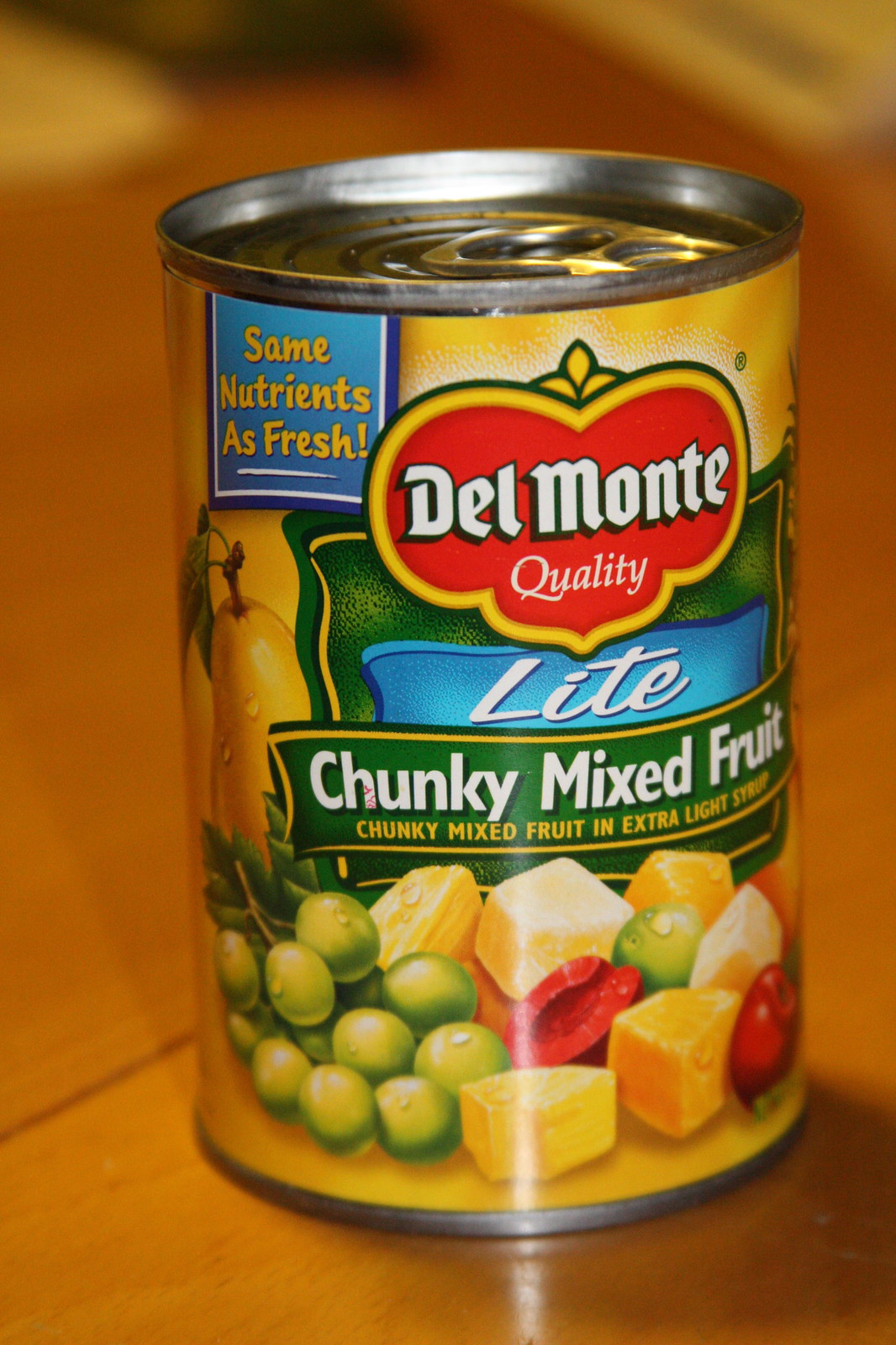The image depicts a can of Del Monte Chunky Mixed Fruit placed on a light brown wooden table. The can features a silver top with a pull-tab, making it easy to open without a can opener. The label on the can is prominently centered, showcasing vibrant colors and an organized layout. At the top left of the label, written in yellow text within a blue background, it says, "Same nutrients as fresh." The brand "Del Monte" appears centrally in white text against a red background, outlined in yellow, with "quality" written beneath it.

Below that, the word "light" is displayed in white text on a blue rectangular background. Further down, the phrase "chunky mixed fruit" appears twice: once in white text within a green ribbon-shaped box with yellow borders, and again in yellow text stating, "chunky mixed fruit in extra light syrup." The bottom section of the label features animated images of various fruits including green grapes on the left, pineapple chunks, cherries (one of which is cut open), yellow pears with green leaves, what appears to be papaya and peaches. This assortment of fruits vividly decorates the label, emphasizing the mix of contents in the can.